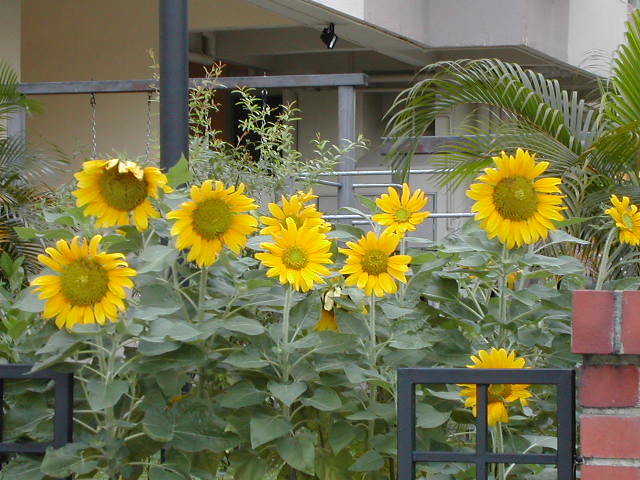The image captures a vibrant outdoor scene in a metropolitan area, featuring a lush garden against the backdrop of an apartment building. The garden is alive with fully-grown, bright yellow sunflowers, whose heads tilt slightly forward, revealing a mix of yellowish-green centers and green leaves at the base of their long stems. Interspersed among the sunflowers are smaller lilies, adding to the floral variety. The garden is enclosed by a black-painted metal fence, with another fence visible further behind. In the bottom corners of the photo, brick banister columns and a metal gate add architectural interest. In the background, we see a white concrete building adorned with metal banisters and chains, possibly part of a swing set, along with gray panels. Suspended from one of the rafters is an outdoor light fixture that resembles a security camera. Adding to the greenery, palm tree leaves and various bushes enhance the scene's lushness, while a few black chairs or window guards rest by a brick wall, completing the urban garden setting.